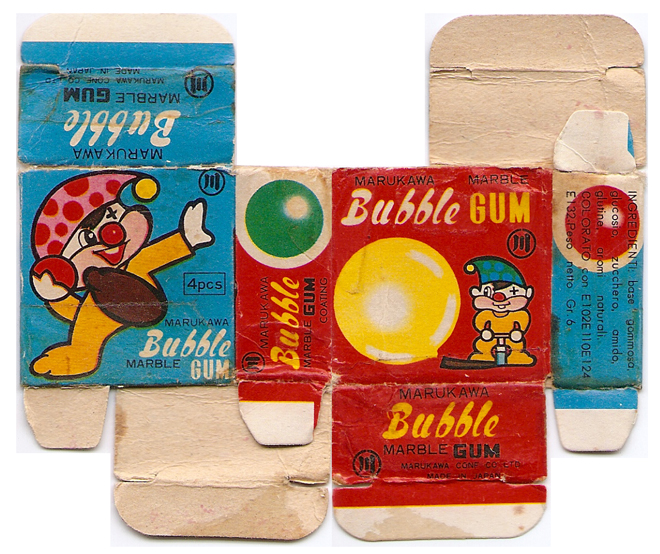This is a color photograph of a flattened Marukawa Marble Bubblegum box, presented on a background that appears white-gray. The packaging has been meticulously taken apart and laid flat to reveal all sides of the box in a single overhead shot. The box is predominantly red and blue, adorned with vibrant cartoon illustrations. Prominently featured is a clown-like mascot with a blue and green hat and a yellow jumpsuit, depicted in playful activity—using a tire pump to inflate a bubblegum ball on the front, and seen throwing a ball elsewhere on the box. The gum balls depicted are a variety of colors, including yellow, green, and red. The box also details that it contains four pieces of gum.